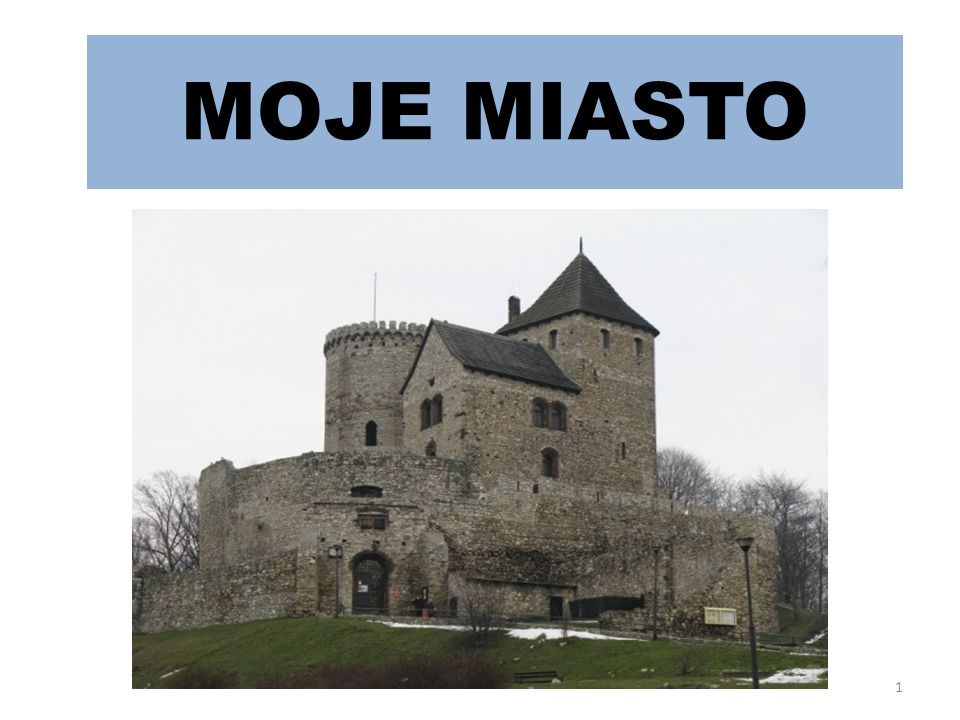The image portrays a stone castle with a prominent tower and a greyish slate roof. The castle, resembling a large townhome and standing approximately two to three stories high, is set amidst a green lawn. Adding to the historic feel are the bare trees around it, indicating late fall or early spring. A pathway leads to the front entrance, flanked by a streetlamp and a small, unreadable sign in the lower right corner. The sky is completely overcast, casting a grey hue over the scene. Above the castle, a blue rectangular banner with the black text "M-O-J-E-M-I-A-S-T-O" can be seen. There are small patches of snow still visible on the grass, emphasizing the wintry atmosphere.